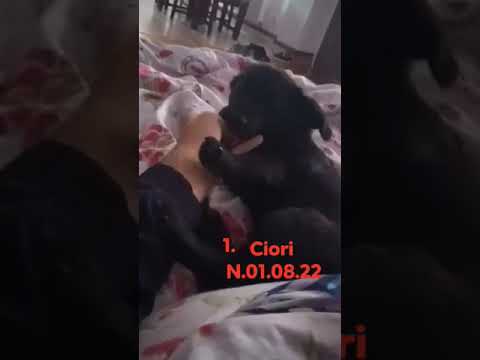The image features a small, black-coated puppy with floppy ears and big paws. The puppy is centrally positioned, slightly to the right, with its paws wrapped around a peach-colored hand, which seems to be its owner's. The owner’s sleeve is partially visible and is black. The puppy and hand rest on a white and pink blanket that covers approximately the bottom three-fourths of the image. The background showcases a light wood floor that occupies the top quarter of the frame. The text "1Ciori" in red font, followed by "N.01.08.22", is displayed over the dog's leg. The overall setup suggests that the photo was taken with a smartphone, possibly for a social media post, as indicated by the black borders on the left and right sides. The scene might be set on a bed, inferred from the floral pattern on the blanket and the positioning of the hand and puppy.